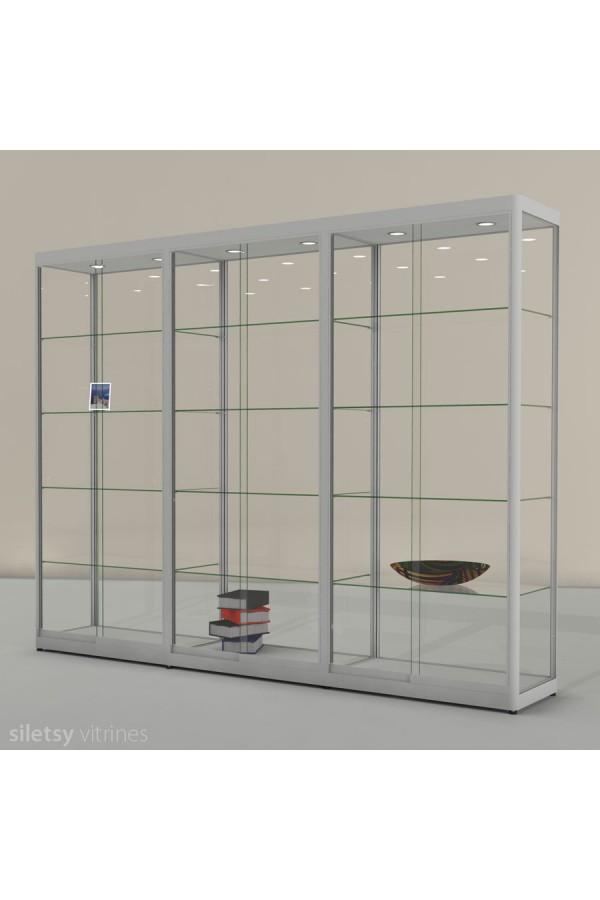This photograph showcases a tall, rectangular glass cabinet with white framing and trim, positioned against an off-white wall and standing on a light gray floor. The cabinet is divided into three vertical sections, each featuring four glass shelves, plus the bottom surface. The glass sliding doors enhance its elegant, modern aesthetic. The interior lighting includes six white light pods embedded in the top, illuminating the contents neatly organized within the cabinet.

On the bottom middle shelf, there is a stack of four hardcover books, arranged in varying directions. The books are distinguished by their colors: dark blue, black, red, and another dark blue or black volume. The right section’s second shelf from the bottom holds a wide, flat wooden bowl, showcasing a predominantly brown and black coloration, possibly with an Egyptian or African design. Meanwhile, the third shelf from the bottom on the left section features a framed photograph with a white border, likely depicting a blue-hued landscape or beach scene. The angled presentation of the shelves subtly faces left, creating a dynamic visual display. Lastly, the words "Siletzi Vitrines" are inscribed in light gray text at the bottom left of the image.